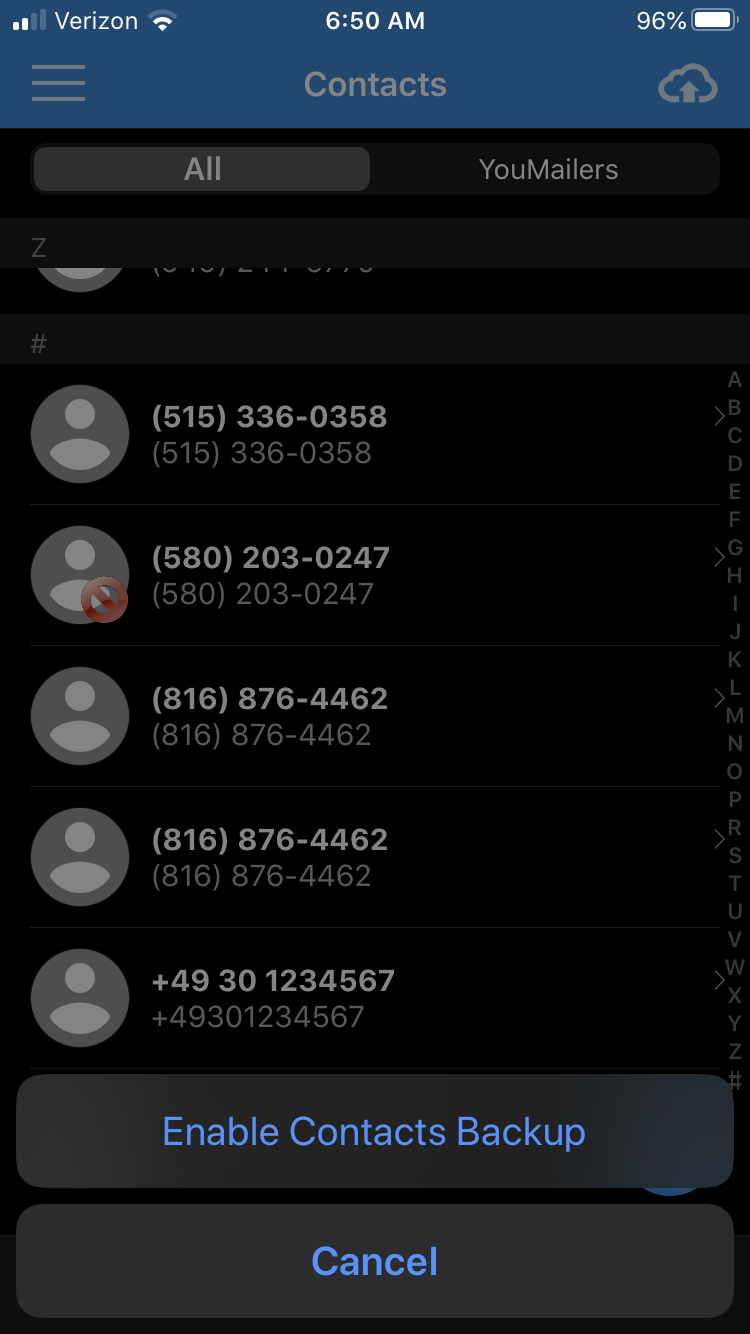**Caption:**

The image depicts a smartphone screen displaying a contacts management application. The interface follows a vertical layout characteristic of smartphone screens.

- **Top Bar:**
  - On the top left, the status bar indicates a Verizon network connection with the Wi-Fi symbol beside it.
  - Centered on the top, the current time is displayed as "6:50 AM."
  - On the top right, a battery icon is displayed at 96% charge.

- **Main Interface Header:**
  - Below the status bar, a blue header displays the word "Contacts" in the center.
  - On the left side of this header, there are three stacked white bars, which likely represent a menu icon.
  - On the right side, a cloud symbol with an upward-pointing arrow suggests an upload option.

- **Contacts Management Area:**
  - The black section below the header features two tabs labeled "All" on the left and "You Mailers" on the right. "All" is highlighted in gray.
  - Beneath these tabs is a segmented list starting with the letter "Z," indicating contact grouping by alphabetical order.
  - The list includes contacts represented by gray placeholder icons, with associated phone numbers:
    - 515-336-0358
    - 580-203-0247
    - Three additional contacts follow in a similar format.

- **Bottom Buttons:**
  - At the bottom, two large gray buttons offer options:
    - "Enable Contacts Backup"
    - "Cancel"